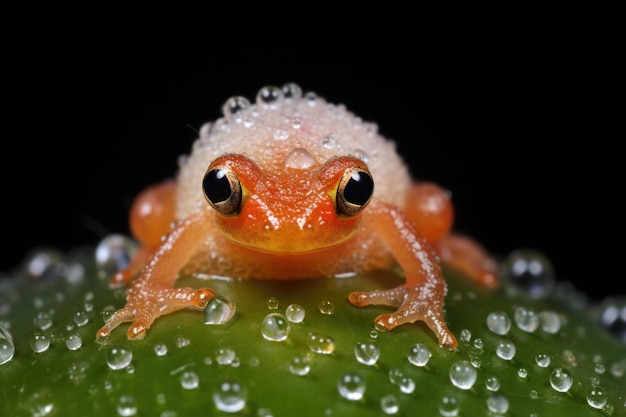In this high-quality, color photograph, the subject is a small, orange toad centrally positioned on a green leaf, which is adorned with numerous glistening water droplets. The toad, detailed with big, bulging eyes that are black with gold borders, appears to be facing the viewer directly. The toad’s head is adorned with clear, almost white bubbles, resembling soap bubbles. The mouth is a simple horizontal line with a subtle hint of yellow above it. Clearly visible are his two front feet, each with three elongated toes. The image is set against a stark black background, accentuating the vivid colors and fine details of the toad and the leaf.